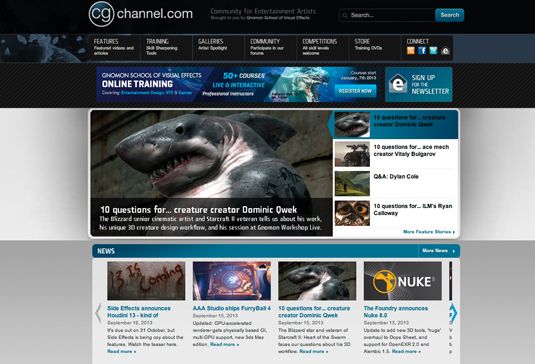This image displays a well-structured webpage layout for an entertainment artist community site.

Starting from the top, there is a thick top border, approximately one inch in height. Positioned about two inches from the left edge, there is a prominent blue circle with a grey border and filled with grey shading. Inside the circle, the letters "CG" are displayed. To the immediate right of this circle, the text "channel.com" is presented in grey.

Below this main heading, a smaller grey text reads "community for entertainment artists." There is also some additional small lettering that is too blurry to decipher. Adjacent to the right side of this text, a search bar is visible. The search bar contains the word "search" written in white text. To the right of the search bar, there is a blue tab with the word "search" also written in white.

Below this header section, there is a light blue border running horizontally across the page, containing seven black tabs separated by grey lines. These tabs, labeled with white text, are "features," "training," "galleries," "community," "competition," "store," and "connect." Each tab has descriptive words underneath, except for the last tab, which includes four social media icons—Facebook, Twitter, and two others that are not clearly identifiable.

The main body of the page features an advertisement for online training. Adjacent to this, on the right side, there is a square box inviting users to "sign up for the newsletter."

Below this area, a large visual element is a picture of a shark that spans about two-thirds of the page width. Underneath the shark image, a headline reads: "Ten Questions for... Creature Creator Dominic Owen," followed by two underlines. To the right of this section, there are four clickable rectangles, each with images on the left and corresponding information in black text on the right. The top rectangle features a blue overlay.

Lastly, at the bottom section of the layout, there is a thin blue border. On the left side, it says "news" in white text, and on the right side, "more news," also in white. Below this border, the page is organized into four rows, each displaying a picture on top with related information underneath.